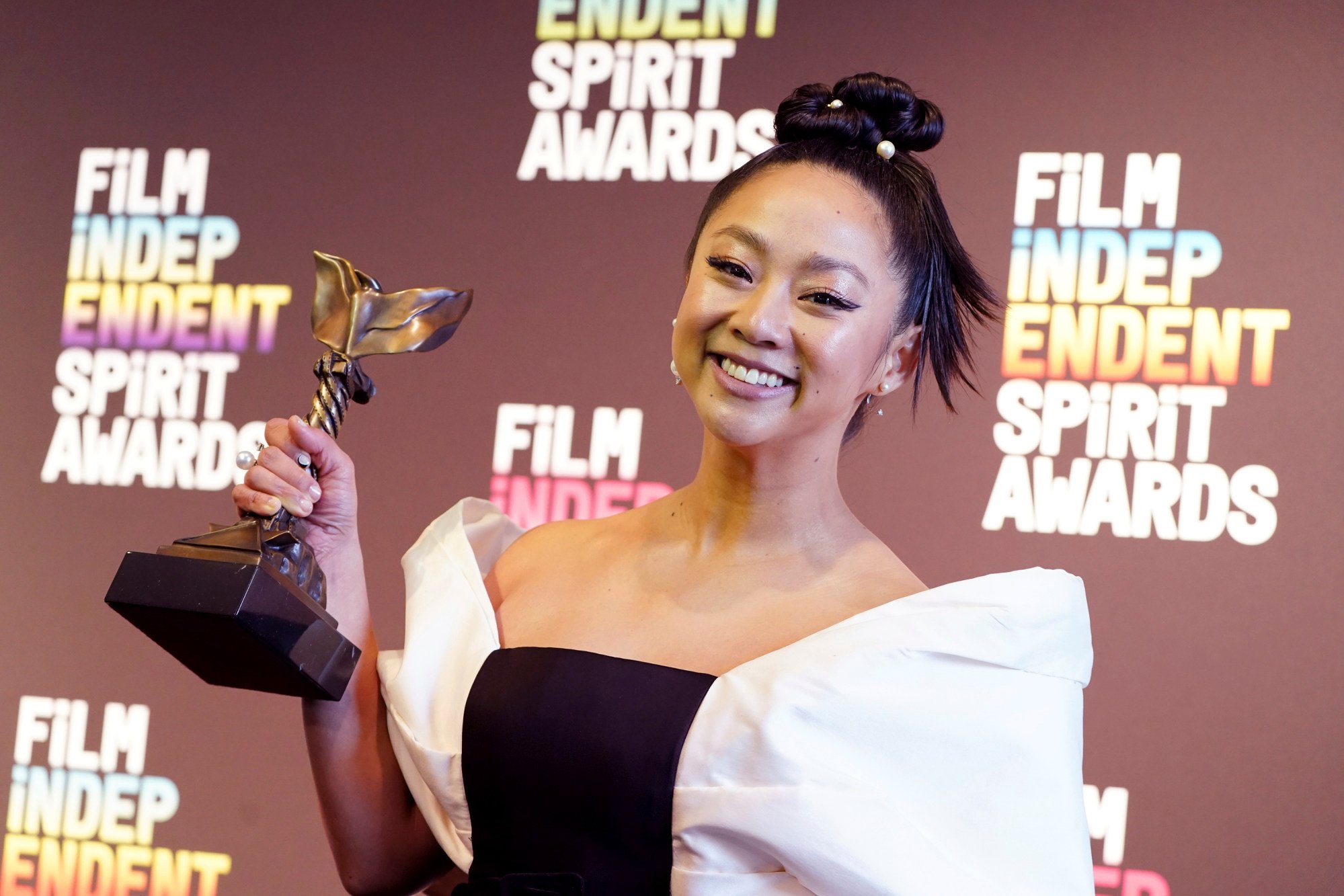In this color photograph, an Asian woman is captured at the Film Independent Spirit Awards. She stands against a mauve backdrop that prominently displays the event's name in a colorful pattern: "Film Independent Spirit Awards" in varying hues of white, pink, yellow, and purple. Her dark hair is styled into a high bun adorned with pearl accessories, and she smiles brightly, showcasing her teeth.

Her outfit is a striking ensemble featuring a black sleeveless dress complemented by large, billowy white off-the-shoulder sleeves. The dress accentuates her bare shoulders, adding a touch of elegance to her appearance. In her right hand, she proudly holds a bronze-colored award with a distinctive whale-tail shape at the top, supported by a pillar and a dark brown wooden base.

The photograph focuses on her from the chest up, capturing her jubilant expression and the intricately designed award she has received. The image beautifully encapsulates her moment of triumph at the event.